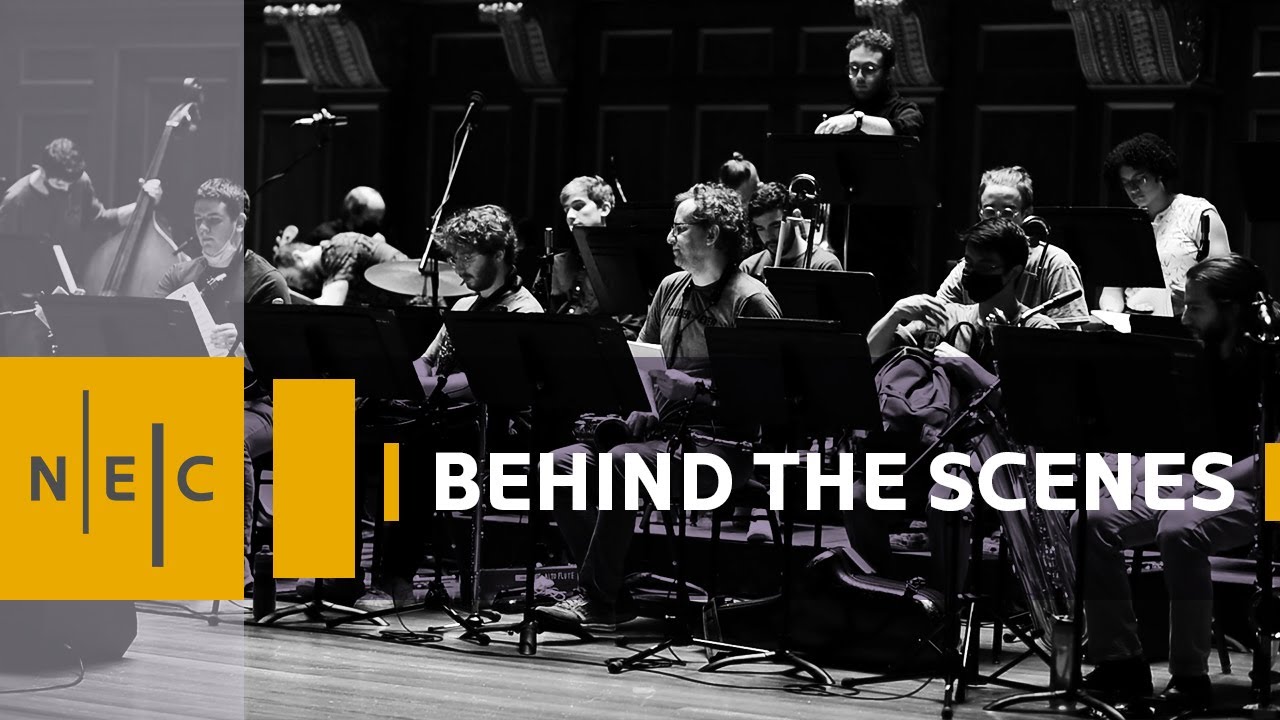The black-and-white photograph captures a candid, behind-the-scenes moment of an orchestra during a practice session. In the image, approximately three rows of musicians are casually dressed, indicating a rehearsal environment. To the left, in all capital letters, the text BEHIND THE SCENES is prominently displayed, while a logo with the letters "N.E.C," separated by vertical lines, is positioned nearby, possibly signifying an organization or broadcasting channel. One notable musician on the left holds a cello and is wearing a mask, reflecting contemporary health precautions. Another individual on the right is seated with a backpack. A man stands at a podium in the background, likely the conductor, guiding the ensemble. Music stands, wires, and sound equipment are scattered across the stage, adding to the authentic feel of the practice setting.